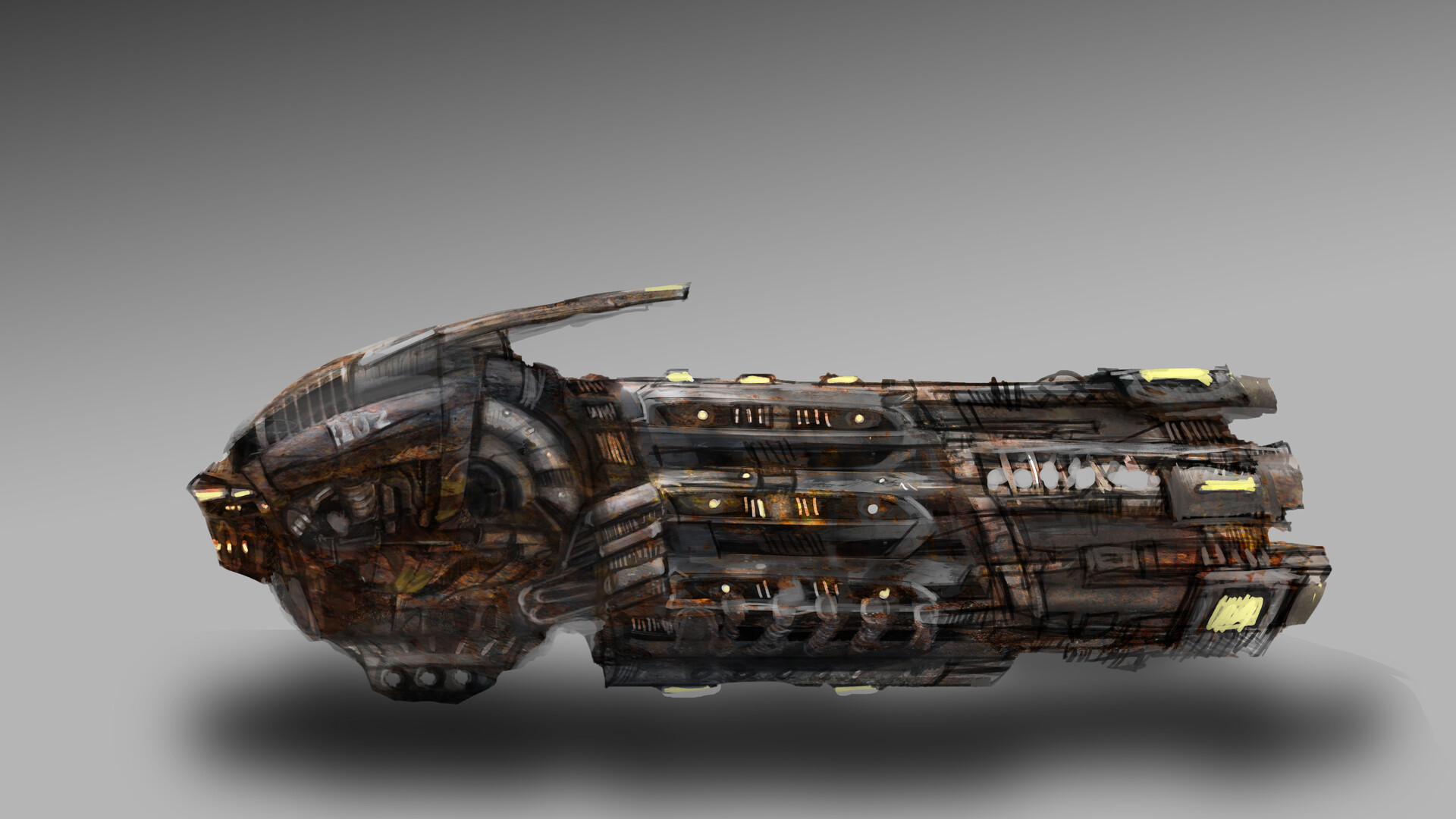The image depicts a detailed drawing of a futuristic hover bike. The hover bike is small and metallic, predominantly brown with amber-yellow lights accentuating various parts of its structure. The front of the bike features a round shape with a flared windshield that curves backward. There is a distinctive round base with gray dots, likely representing a hover engine. Toward the middle, the bike has a hand rest or handlebar on the left side. The cabin area is gray-silver metal, curved and tubular, merging into the brown center portion, which includes a brown headlight grill and amber glowing lights. The rectangular rear section houses a large engine flanked by squared light panels with horizontal yellow lights and gray tubes connecting different parts of the bike. Additionally, yellow lights are visible on the top of the bike. The entire vehicle casts a gray drop shadow on the light gray background.